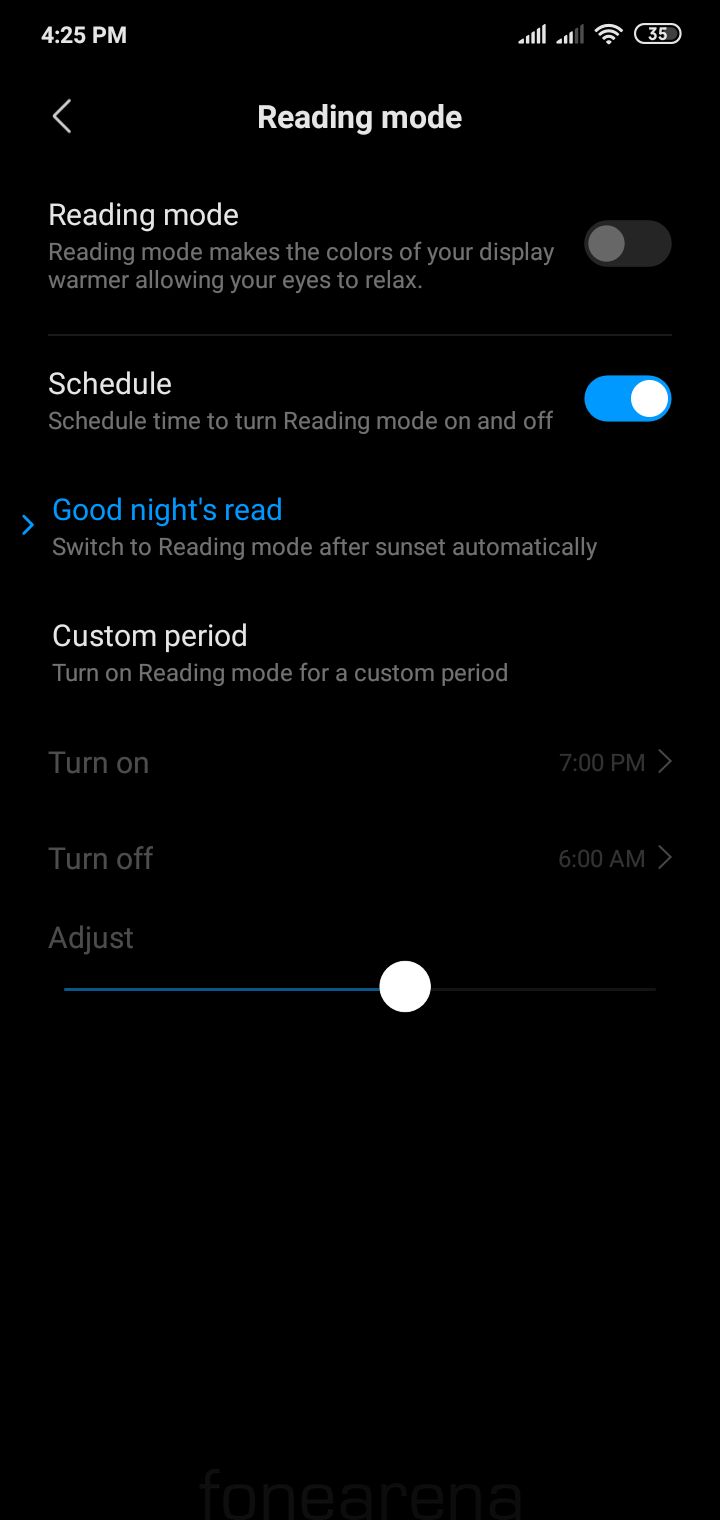The black and white background of the phone screen is adorned with multiple status indicators in the upper corners. On the top left, the time is displayed as "4:25 PM." Adjacent to it on the right, two service bars can be seen; the first bar is completely white, indicating full service strength, while the second bar—with three white bars and two grey ones—suggests a slightly lower signal strength. All the Wi-Fi signal lines are white, indicating a strong Wi-Fi connection.

Central to the display is an interface for toggling Reading Mode. An oval icon with a black center and a white number "35" is present, surrounded by a white outline. Adjacent to this icon is a left-pointing arrow in white. The bold text "Reading Mode" appears prominently, followed by a brief description: "Reading mode makes the colors of your display warmer, allowing your eyes to relax."

Further down, there's a grey circle on the left side within an oval, indicating the option to turn off Reading Mode. A white line crosses through this circle. Below it, the interface shows a scheduled time feature to automatically manage Reading Mode. It is currently set from "7 PM" (start time) to "6 AM" (end time). The scheduled time toggle is blue with a white circle on the right, reflecting that the feature is enabled. Simultaneously, the blue end of an arrow points to the right, reinforcing this status.

Additionally, the interface allows customization with a section titled "Custom Period" for setting specific Reading Mode activation times. Under this, a blue and grey adjustable bar with a white circle in the middle allows the user to fine-tune their preferred start and end times for Reading Mode activation.